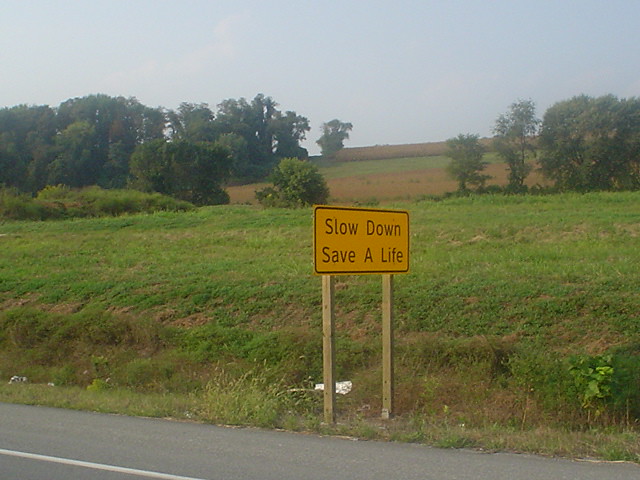A roadside sign stands prominently in the foreground of this picture, taken from a side view. The rectangular, yellow sign, edged in black, conveys an important message in bold black letters: "Slow Down, Save a Life." It is supported by two slender wooden posts planted in a small ditch beside the highway. The edge of the road is marked by a white line separating the concrete shoulder from the wild, overgrown grass that forms the ditch. The background rises slightly into a hill covered in a mix of green and brown grass, dotted with shrubbery and trees. Some white litter, possibly a plastic bag, is visible near the sign. The sky above is a clear, uninterrupted blue, providing a serene contrast to the bustling road.